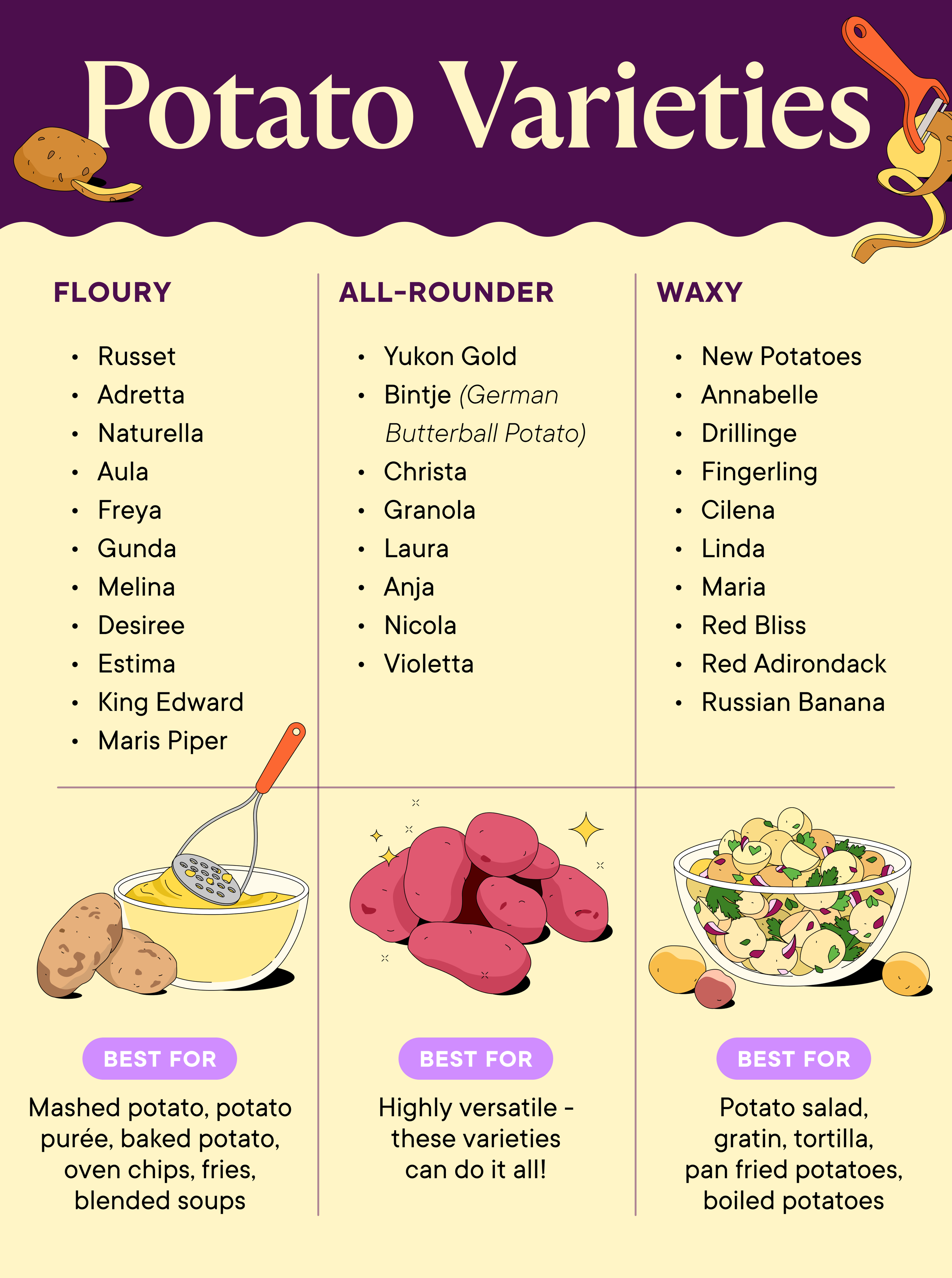The image is a detailed chart differentiating various potato varieties with a vibrant and artistic design. At the top, there's a wide purple banner titled "Potato Varieties," flanked by illustrations of a cut potato on the left and a peeled potato on the right, all set against a decorative black squiggly background. Below this, the chart is divided into three vertical sections, each representing different potato categories: flowery, all-rounder, and waxy. 

The flowery section lists varieties such as russet, freya, and gunda, accompanied by an image of mashed potatoes. The all-rounder section names varieties like Yukon gold, granola, and laura, illustrated with whole red-skinned potatoes and described as versatile for all dishes. The waxy section includes fingerling, maria, and red bliss, with an image of a potato salad emphasizing their suitability for such dishes. Overall, the chart employs artistic clipart to educate viewers about the diverse types and uses of potatoes.